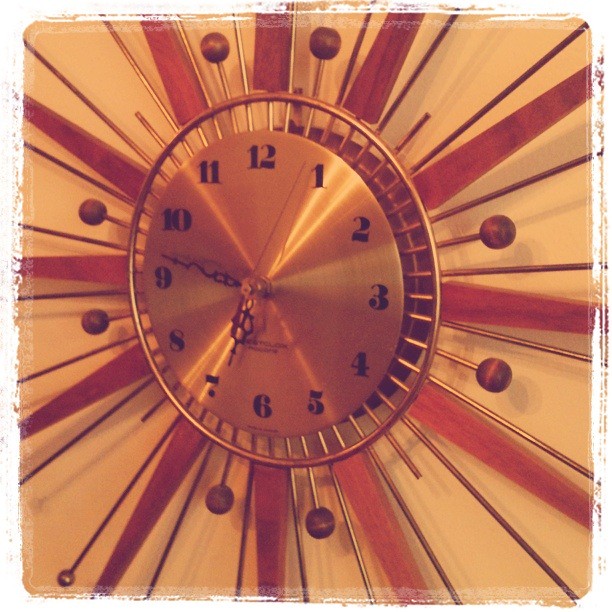This photograph captures a clock designed to resemble a shining sun. The central face of the clock, made of metal with a copper color, prominently features black numerals and two hands pointing to approximately 6:46. Encircling the clock face is a gleaming, solid gold plate, adding to its opulent appearance. From this central structure, numerous metal rods extend outward, each topped with small, globe-like spheres colored in copper and brown. These rods are interspersed with dark-colored wooden rays, creating an alternating pattern that enhances the sunburst effect. The overall composition of the clock, with its orangish-yellow hue and shiny brass-like elements, is further accentuated by the glare reflecting off its surface. The image itself is taken at a slight angle, with the right side appearing closer than the left, and has a border that fades out, resembling a painting.